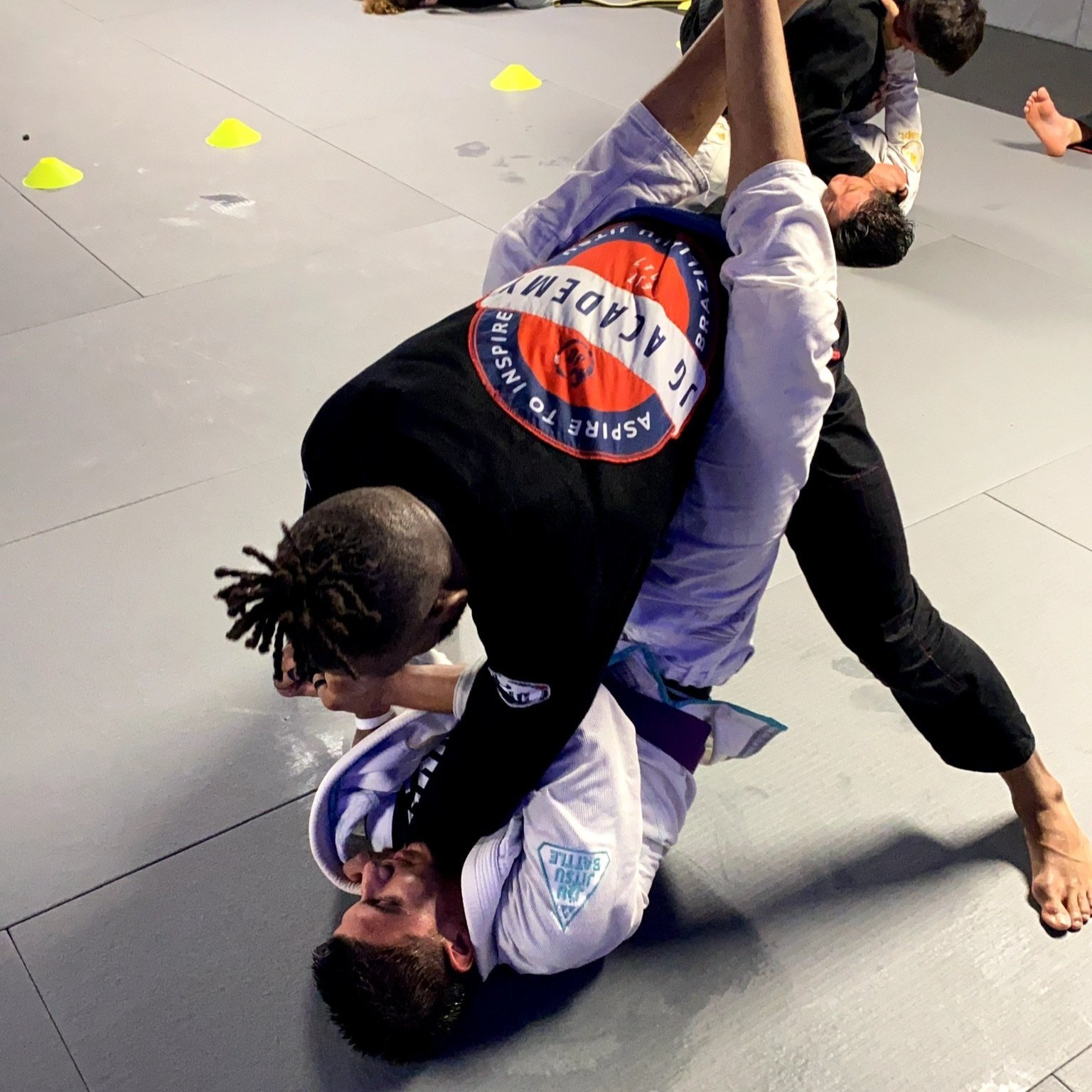The photograph depicts a jiu-jitsu training session, with a focus on two primary practitioners in the foreground. The individual on top, wearing a black gi with a circular patch on his arm and bright hair, is crouched over a man in a white gi who has locked his legs around the former's waist while securing a body lock. Additionally, the man in white is controlling the arm of his opponent, who has his arm pressed against the white gi wearer's neck. Both participants have black hair. In the background, more students are practicing jiu-jitsu on a white-tiled floor with some black tiles towards the top right corner. The setting is a jiu-jitsu academy, demonstrated by the branded outfits of the trainees. Among those in the background, some are engaged in their own drills while others may be seated, partially visible with their feet on the mat. The image captures an intense and detailed scene of martial arts training.